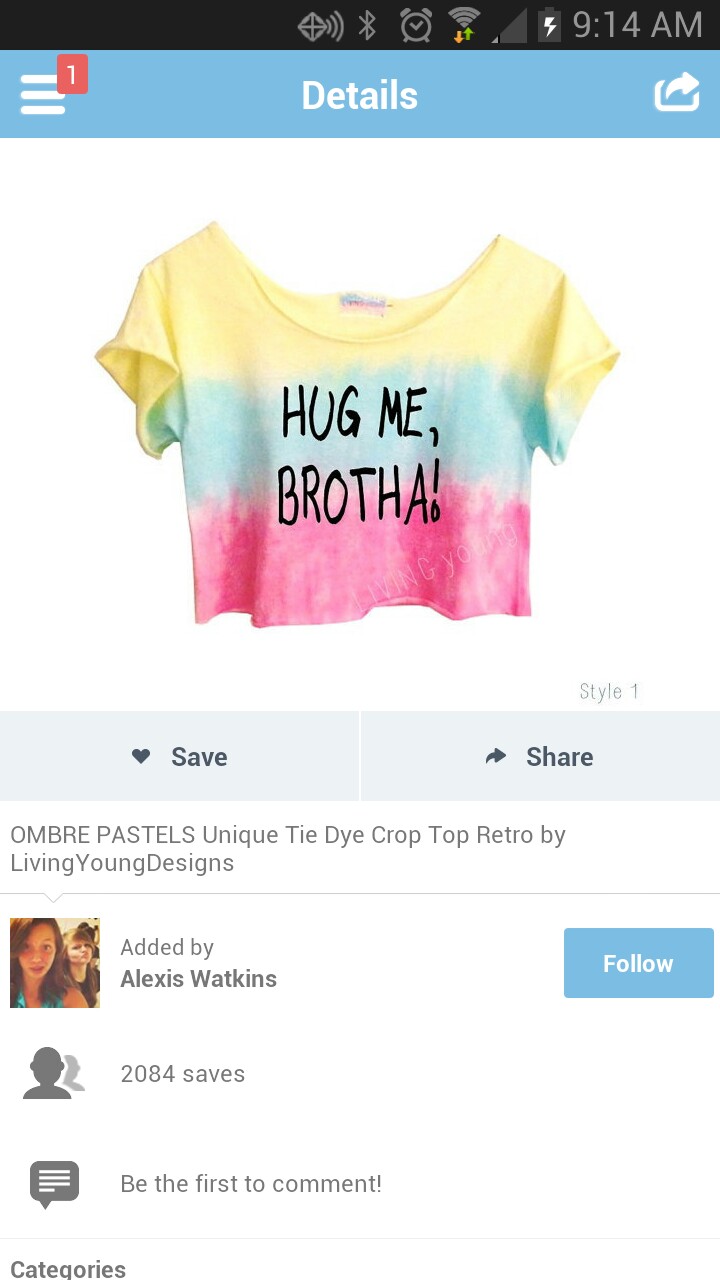The image is a phone screenshot showcasing an online store listing for a crop top shirt. The phone’s status bar, visible at the top, displays various icons including Bluetooth, alarm, Wi-Fi, and a charging battery, with the time marked as 9:14 AM. A light blue horizontal bar beneath the status bar reads "Details" in white text. The shirt featured prominently in the center of the screen is a colorful crop top with yellow at the top, blue in the middle, and pink at the bottom. Bold black text in the middle of the shirt reads, "Hug me brother!" On the left-hand side beneath the shirt is a "Save" button, and to the right, a "Share" button. Below this section, the product description reads, "Ombre pastels, unique tie-dye crop top, retro by Living Young Designs," followed by the line, "Added by Alexis Watkins." There’s a blue "Follow" button to the right. The listing mentions the shirt has 2,084 saves and invites users to "Be the first to comment."